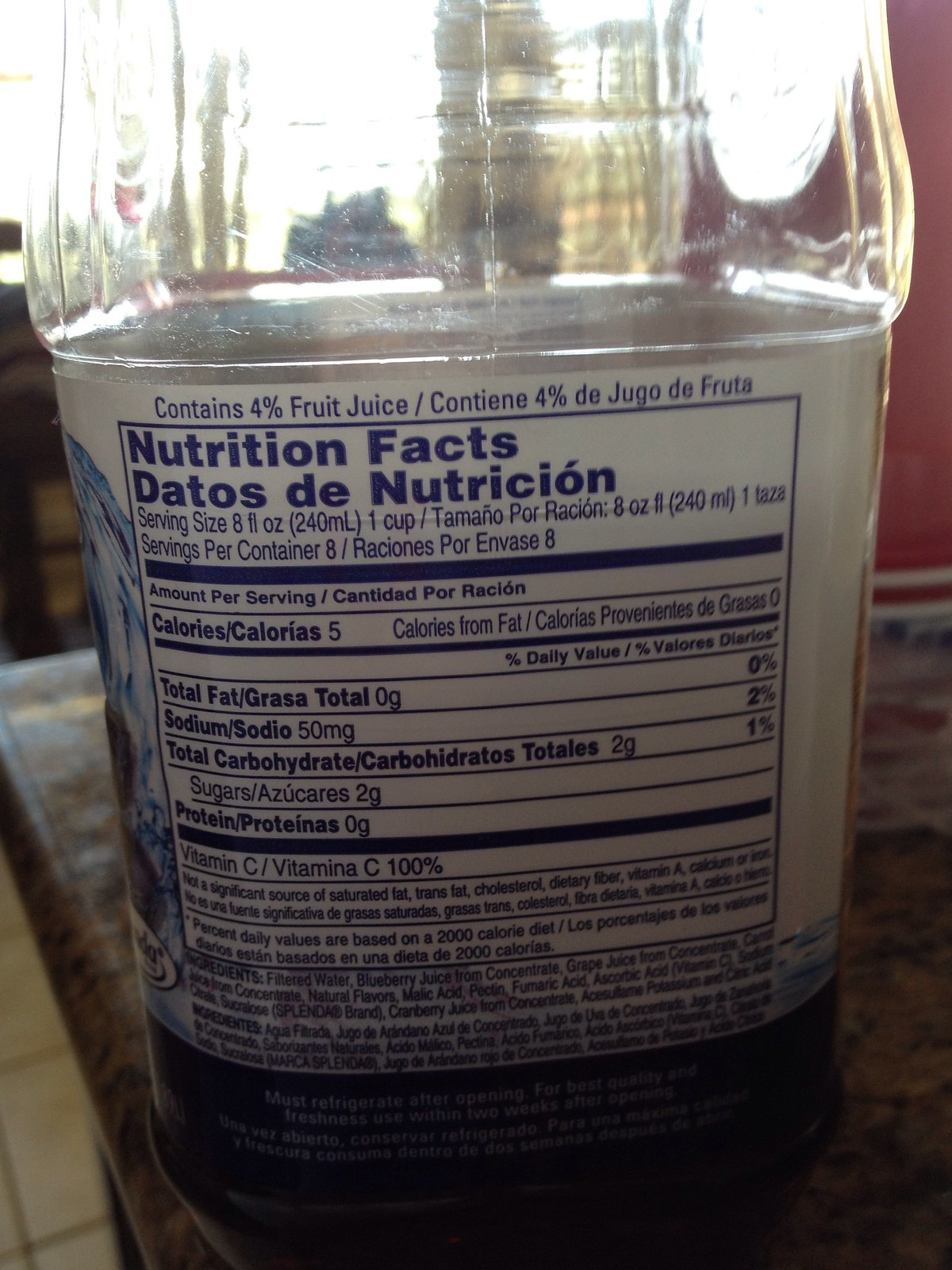The image captures a vertically rectangular, close-up view of a large plastic juice bottle with rounded edges but an overall rectangular shape. The focus is on the back of the bottle, which features a white label adorned with a blue nutritional facts box. Above the nutritional information, a clear statement reads "Contains 4% juice." The serving details are specified as "Serving size: 8 fluid ounces" and "Servings per container: 8." The nutritional facts box includes comprehensive details such as calories, total fat, sodium, and other nutritional content. The upper part of the bottle is transparent, devoid of any labeling, revealing the liquid inside.